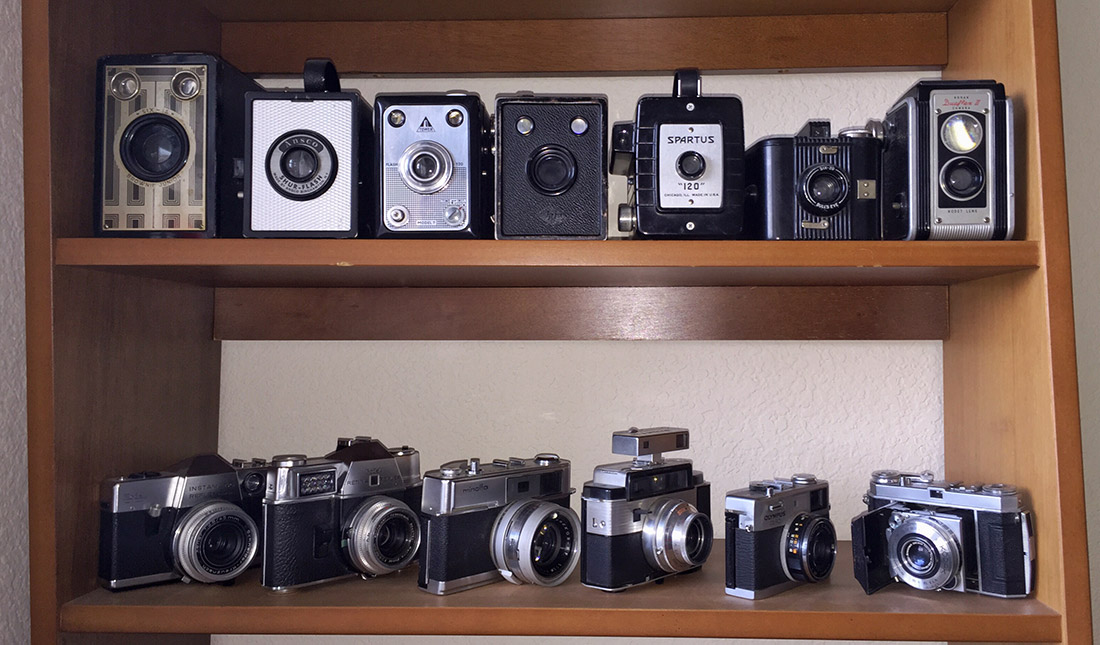This image showcases two brown wooden shelves fixed against a white wall, each adorned with an array of vintage cameras. The top shelf features earlier vintage models that are boxy and robust, with several bearing names like Spartus and Flash, hinting at their age and possibly serving as projector cameras or moving picture cameras. These cameras predominantly exhibit a classic black and silver color scheme, with a noticeable rectangular front design. On the lower shelf, the cameras, though still vintage, are relatively more contemporary. There are six cameras in total, each equipped with adjustable lenses extending outward. They display a consistent design aesthetic: the lower part of the camera housing is black, while the upper parts flaunt a metal or brushed metal finish. Among these, one camera stands out with a unique top extension, adding to the eclectic mix of this photographic collection.